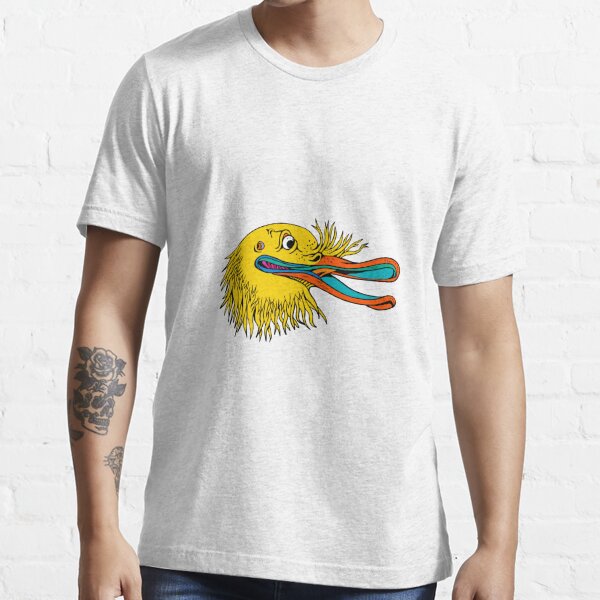The photograph features a man standing upright against a white brick wall. He is wearing a short-sleeved, off-white t-shirt adorned with a detailed drawing of a duck's head. The duck has a yellow face, an orange beak with a teal interior, and an angry-looking eye. Its head is surrounded by scraggly feathers above and below the beak. The man is also dressed in blue jeans, although only a small portion of the jeans is visible as the photo cuts off at the hips and upper legs. Prominently, he has a rose tattoo in dark black ink on his right arm, as well as another tattoo on his forearm, which is partially obscured in the image.